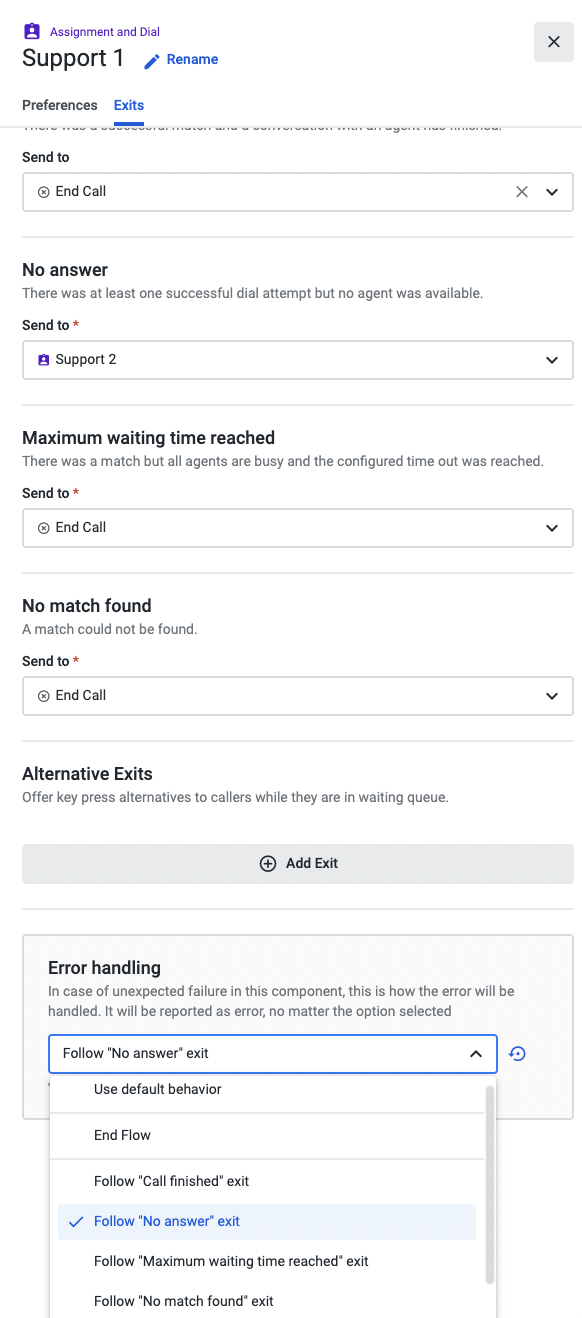This is a detailed caption describing a smartphone screenshot of a web page interface used for handling call assignments and error management. The page begins at the top with a user photo icon next to text that reads "Assign Assignment and Dial," accompanied by a closeout "X" icon on the right. Below this, there is a "Support 1" label and a "Rename" link, followed by "Preferences" and an "Exits" link.

Further down, the page displays a "Send to" section featuring an "End Call" option, which you can close by clicking the closeout cross labeled "X" or use the drop-down arrow to the right. Beneath this box, the page states "No Answer: There was at least one successful dial attempt, but no agent was available."

Next, another "Send to" section features a user profile icon and the label "Support 2" with a drop-down arrow to the right. Underneath, it reads "Maximum Waiting Time Reached: There was a match, but all agents are busy, and the configured timeout was reached."

Following this is another "Send to" section with "End Call" again, featuring a closeout cross "X" and a drop-down arrow. Below this, the page indicates "No Match Found: A match could not be found."

Further down, the page includes "Send to" and another "End Call" box, complete with a closeout cross and a drop-down arrow. Below this, "Alternative Exits: Offer keypress alternatives to callers while they are in the waiting queue" is displayed, followed by a gray box with an addition sign within a circle labeled "Add Exit."

Finally, the page explains "Error Handling: In case of an unexpected failure in this component, this is how the error will be handled. It will be reported as an error no matter the option selected." There is a drop-down box set to "Follow 'No Answer' Exit," accompanied by entries for possible actions: "Use Default Behavior in Flow," "Follow 'Call Finished' Exit," "Follow 'No Answer' Exit" (which is checked), "Follow 'Maximum Waiting Time Reached' Exit," and "Follow 'No Match Found' Exit."